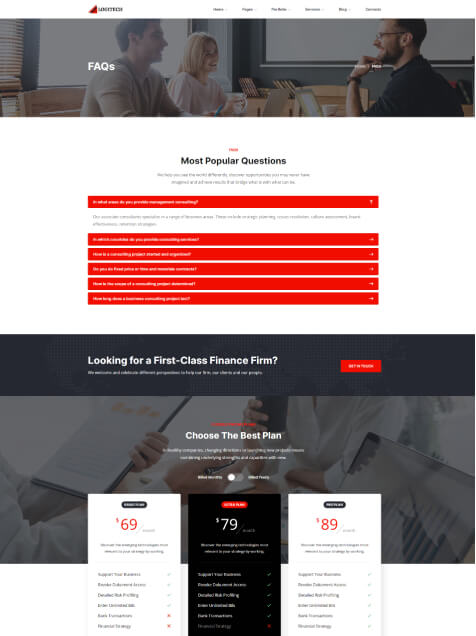This image showcases an extended view of a website, with its content shrunk to fit within a single pane for a comprehensive overview. At the top, the website features a primary navigation menu against a white background, offering six options in general. Below the menu, a banner image depicts three individuals gathered around a table, engaged in conversation, with tablets or laptops in front of them. The group consists of a woman and a man on the left, and another man on the right.

Further down, the page returns to a white background with the section title "Most Popular Questions" prominently displayed in bold, larger font. This title and its accompanying text are center-aligned. The text beneath the title is in a smaller font and is not bold, though it is too indistinct to be readable.

Continuing down the page, there are six horizontally aligned red bars with white text on the left and drop-down arrows on the right. The first bar is expanded, revealing a white background with black text underneath, though the specifics of the text are not visible. The overall layout emphasizes clear sections and ease of navigation through drop-down menus, centering information for a clean and organized appearance.